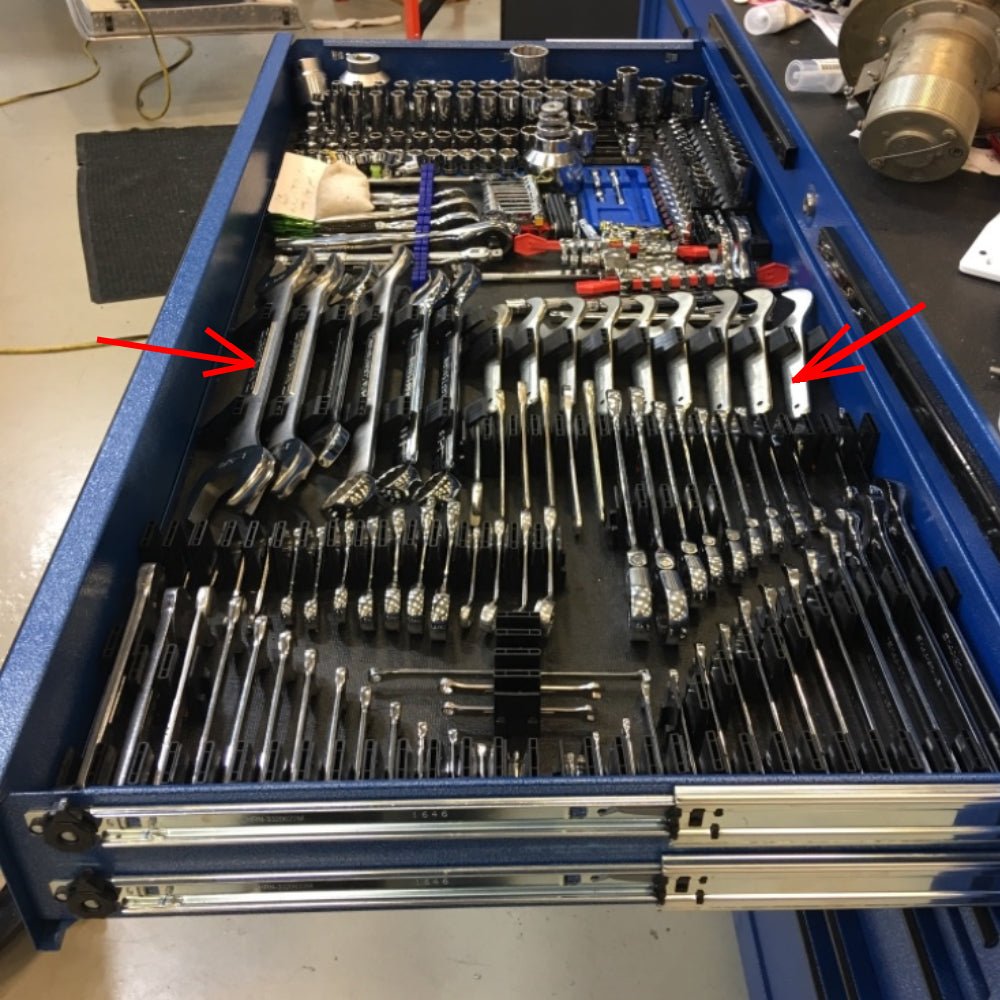This detailed photograph depicts a large, floor-standing blue tool cabinet, specifically focusing on its open top drawer. Inside, the metallic black interior contrasts with the meticulously organized array of silver tools. Predominantly, we see a comprehensive collection of wrenches of various shapes and sizes, neatly arranged in designated slots for easy access. In addition to the wrenches, there are sockets and screwdrivers, some of which feature red handles, further contributing to the well-structured layout. Red arrows, added through editing, point towards the inside of the drawer, drawing attention to the organized placement of the tools. The remaining visible part of the setting includes the ground and additional metallic objects scattered around, adding context to the indoor environment of this highly functional workspace.